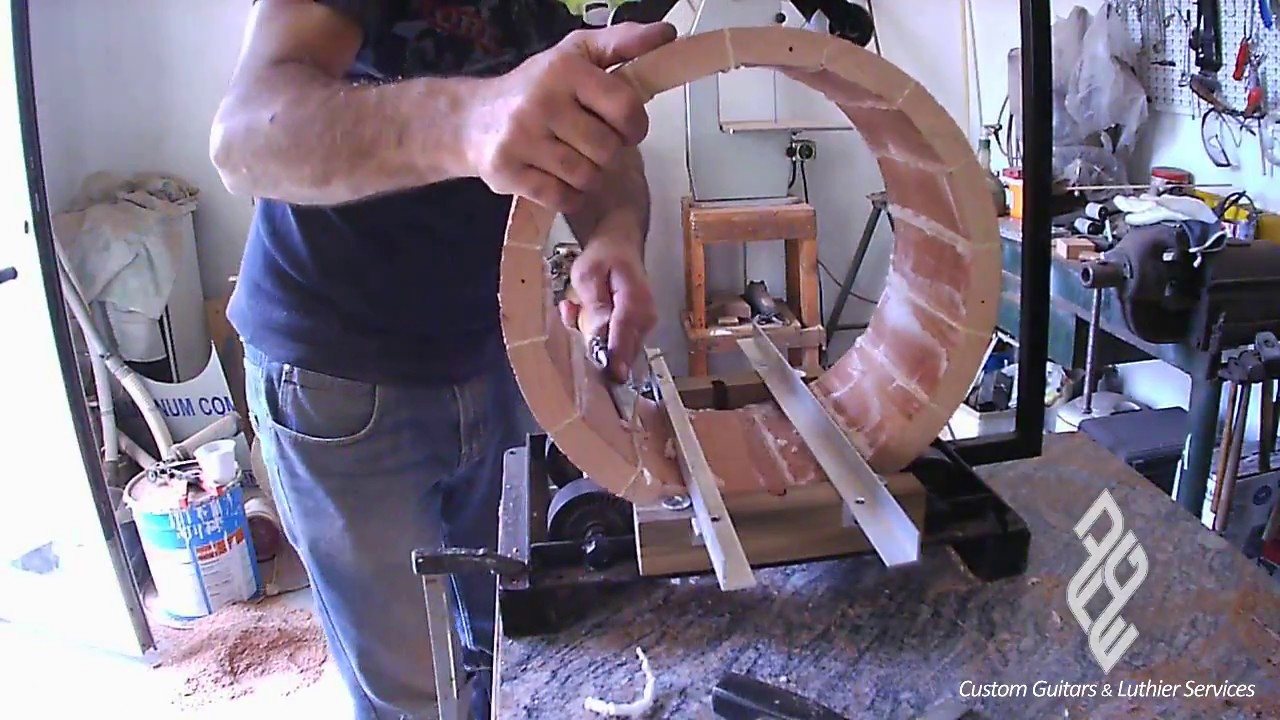In this indoor image, taken in a garage workshop, a man dressed in a blue t-shirt and blue jeans is seen from the shoulders down working on a woodworking project. His head, lower arms, and lower legs are not visible. The man appears to be either sanding or adjusting a circular wooden piece that is securely held by two steel rods and placed on a machine atop a workbench. To the right, tools like screwdrivers are neatly hung on the wall, and another workbench holds several cans and other items. On the left side of the image, an open door can be spotted, along with a can, a bucket with white paint on the outside, and some trash in the corner. Various objects, including bottles and what seems to be a vacuum, are scattered on the countertops in the background. The setting also features a bench running through the work area, enhancing the detailed and busy atmosphere of the man's workspace.